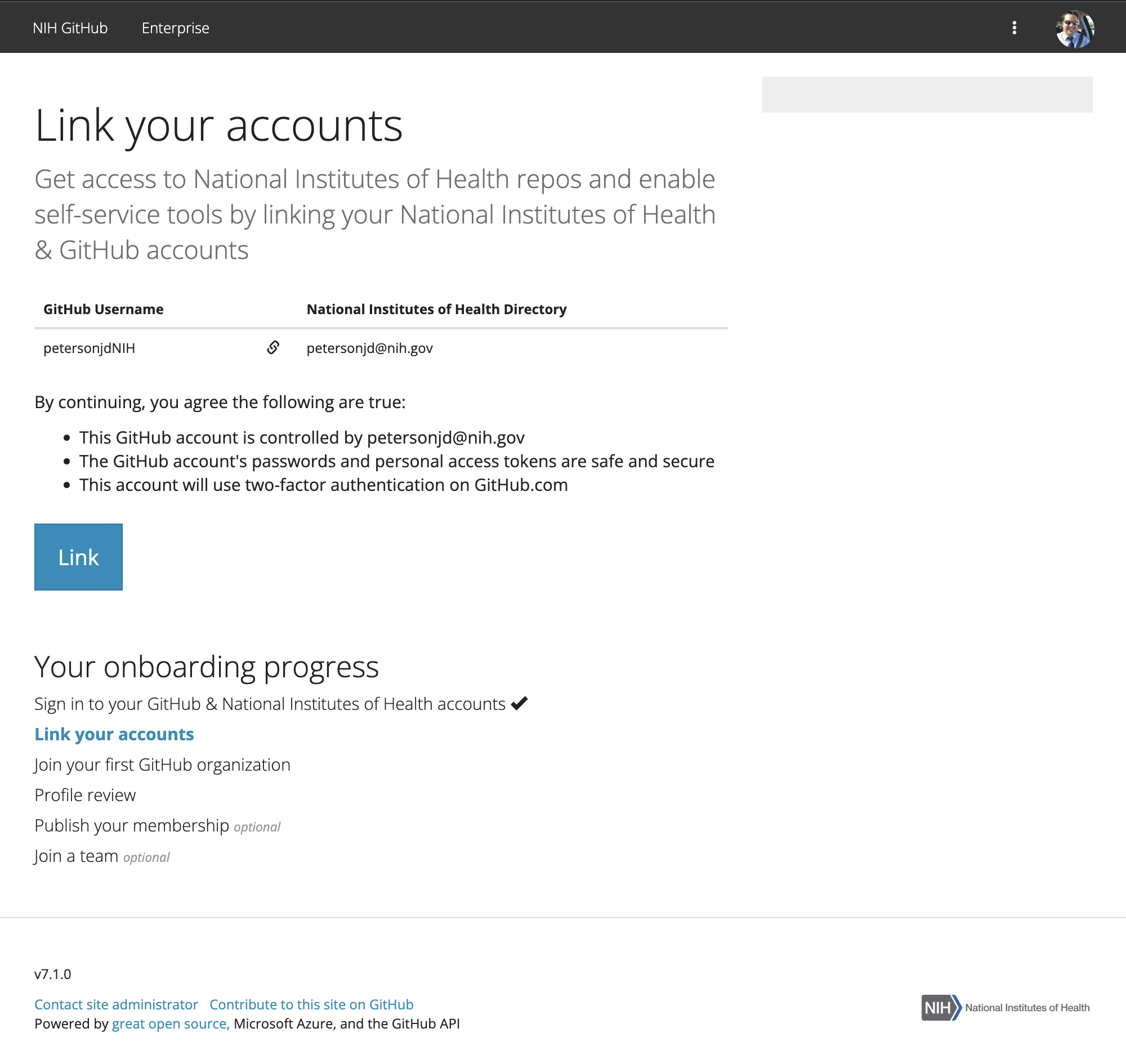**Caption:**

The image depicts a National Institutes of Health (NIH) webpage with a clean, white background. At the top, a black rectangular banner stretches horizontally from left to right. In the left corner of the banner, "NIH GitHub Enterprise" is written in white text. On the right side of the banner, there are three vertical white dots next to a circular image of a Caucasian male. The man has short brown hair, wears glasses, and is dressed in a light blue button-up shirt paired with a dark tie.

Below the banner, on the white background, black text instructs users to "Link your accounts." The text explains that by linking NIH and GitHub accounts, users can gain access to NIH repositories and enable self-service tools.

Following this, there are text fields labeled "GitHub username" and "NIH directory," separated by a gray horizontal line. Below this line, "PetersonJDNIH" and "PetersonJD@NIH.gov" are displayed. An advisory note beneath this states, "By continuing, you agree to the following are true," followed by three bullet points:
1. "This GitHub account is controlled by PetersonJD@NIH.gov."
2. "The GitHub account passwords and personal access tokens are safe and secure."
3. "This account will use two-factor authentication on GitHub.com."

Towards the bottom left, a blue square with white text reads "Link." Further down, a section titled "Your onboarding progress" is listed. The first step, "Sign into your GitHub and National Institutes of Health accounts," has a check mark next to it. Below this, "Link your accounts" is written in blue text. The final steps detailed in black text are "Join your first GitHub organization," "Profile review," "Publish your membership," and "Join a team."